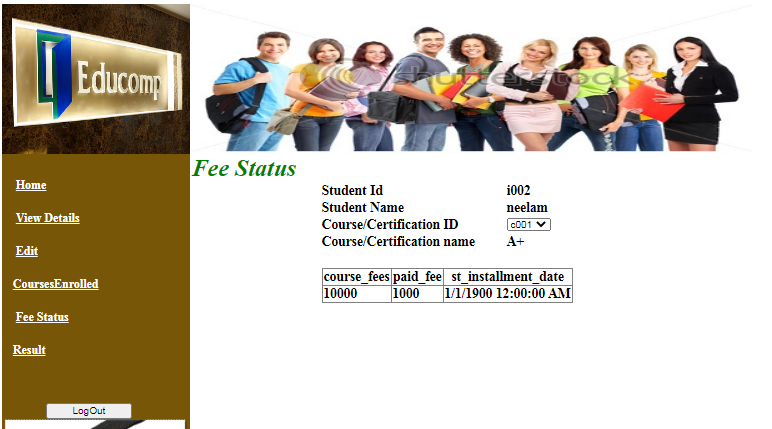The website appears to be a preliminary design for a college management system, presumably under the name "EduComp." The header features a logo consisting of an image of a book accompanied by the word "EduComp." Below the logo, a navigational menu provides links to several sections: Home, View Details, Edit, Courses Enrolled, Fee Status, and Result. A logout button is also present in this section.

Dominating the central portion of the page is an image showcasing a group of models posing as students. Notably, the image carries a "Shutterstock" watermark, indicating it has been improperly sourced and may have been tampered with, as it appears horizontally stretched and distorted.

Below the image, a detailed section in green italic text provides information about a student's fee status. This includes:

- Student ID: I002
- Student Name: NEELAM
- Courses Enrolled with Certification ID: C001
- Course Certification Name: A+
- Course Fees: $10,000
- Paid Fee: $1,000
- Next Installment Date: 01-01-1990 at 12:00 AM

The rudimentary design and various anomalies (e.g., placeholder IDs, improbable dates, and unauthorized image use) suggest that this is either a mock-up or an in-development version of the website. It is likely that further refinements, including the use of legally obtained images, are anticipated before the site becomes fully operational.